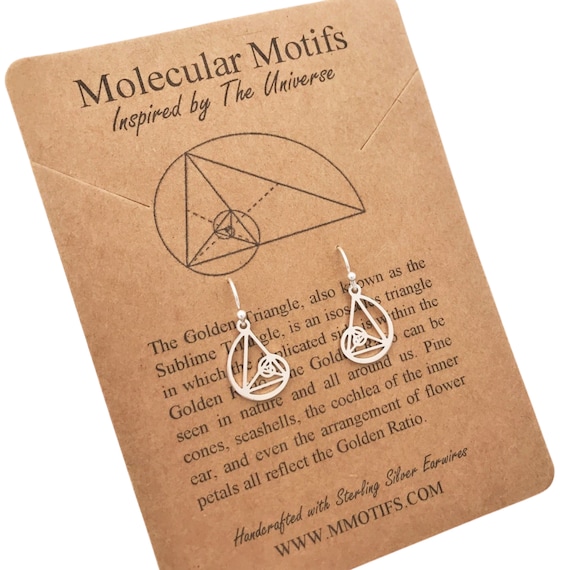This photograph showcases a cardboard earring holder from "Molecular Motifs," featuring a detailed, thematic design inspired by the universe. At the top of the card, "Molecular Motifs" is printed in black font, followed by the cursive text, "Inspired by the Universe." Below this header, there's a sophisticated illustration: a triangle bisected by a line and adorned with a curly Q motif wrapping around the triangle, connecting its points.

The earrings themselves mimic the design depicted above, featuring a stylized triangle combined with a Fibonacci spiral, reminiscent of a nautilus shell or a golden ratio pattern. These earrings are handcrafted from sterling silver, as indicated by the cursive inscription beneath them. The card further provides a brief description of the golden triangle, also known as the sublime triangle, highlighting its connection to the design's mathematical elegance.

Completing the presentation, the website "www.mmmotifs.com" is listed at the bottom of the card, inviting viewers to explore more of these universe-inspired, handcrafted sterling silver jewelry pieces.